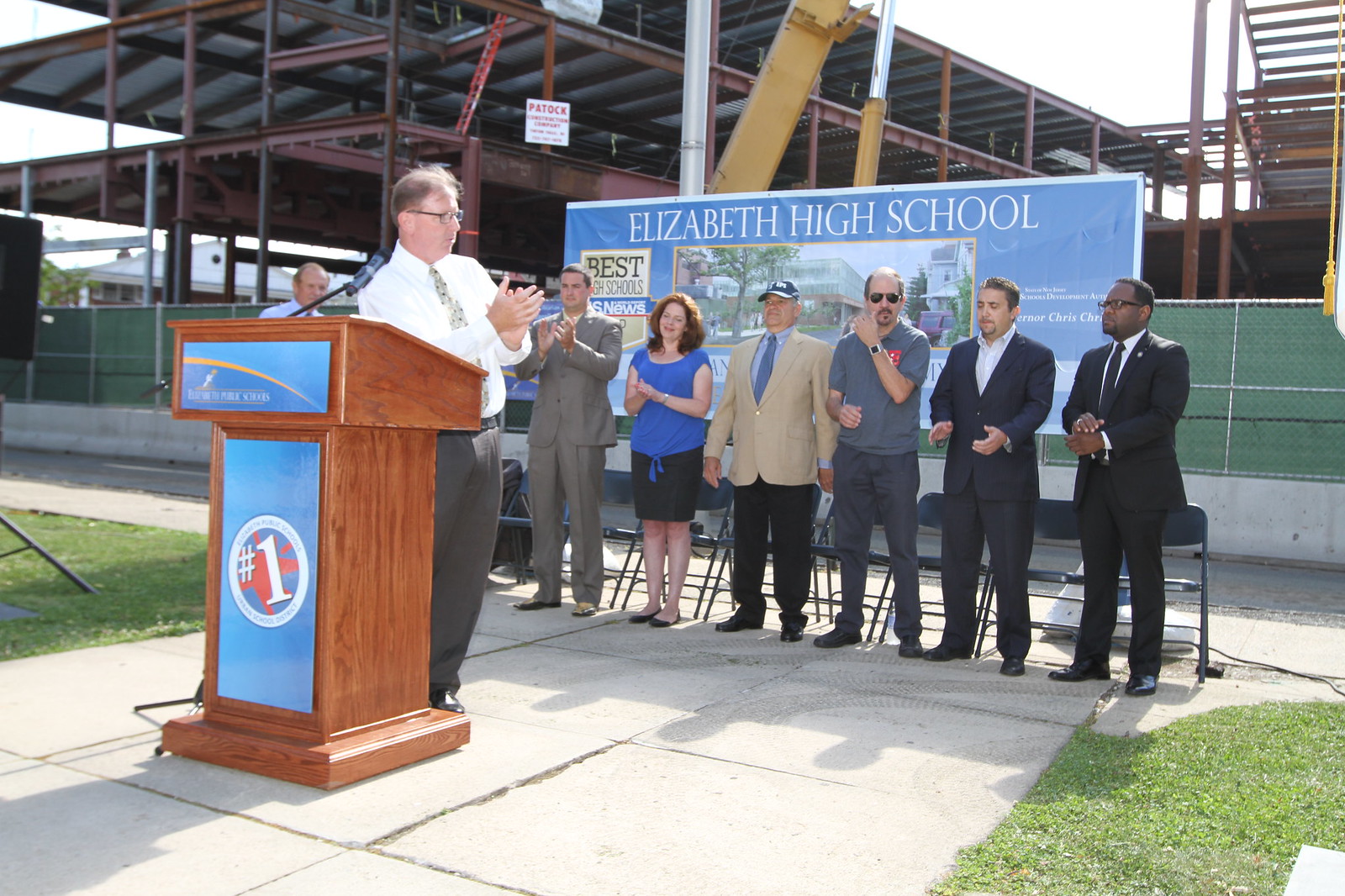The image captures a moment at the groundbreaking ceremony for Elizabeth High School. Central to the scene is a man standing at a wooden podium adorned with a blue sign featuring a white number 1 in a circle. He is wearing gray pants and a white dress shirt, clapping while looking to his right. Surrounding him are seven individuals, a mix of men and women in dress clothing, including suits and skirts. They stand on a cement sidewalk, flanked by green grass, each with a black folding chair behind them. Behind this group, a large blue sign with "Elizabeth High School" written in bold white letters and a rendering of the future school underneath proudly marks the occasion. The sign also highlights a recognition from U.S. News as one of the "Best High Schools." Enclosing the construction area is green mesh fencing, beyond which several floors of the new school’s skeletal structure, made up of steel and red girders, are visible. This setting collectively illustrates the progression and anticipation for the new high school facility.